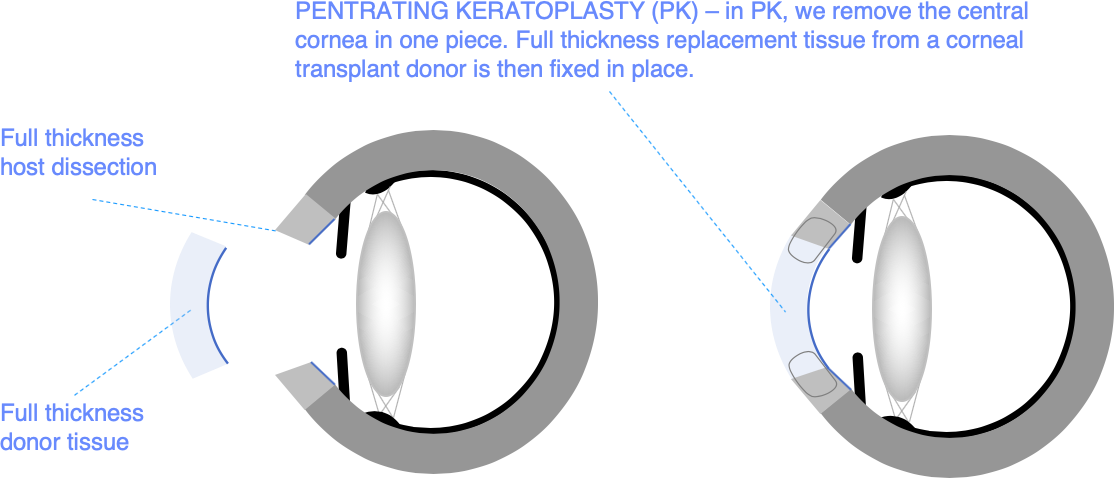This scientific diagram provides a detailed visualization of the penetrating keratoplasty (PK) procedure. At the top, in blue lettering, it explains that the central cornea is removed in one piece. The diagram contains two images depicting the eye from a side view: the first image illustrates the full thickness host dissection and the removal of the cornea. The second image shows the placement of full thickness replacement tissue from a corneal transplant donor. Both images feature the eye represented as a grey circle with a black interior border and a white oval. Notably, annotated lines highlight the areas of dissection and the placement of the donor tissue. The text provides further clarity, stating, "In PK, we remove the central cornea in one piece, and full thickness replacement tissue from a corneal transplant donor is then fixed in place."